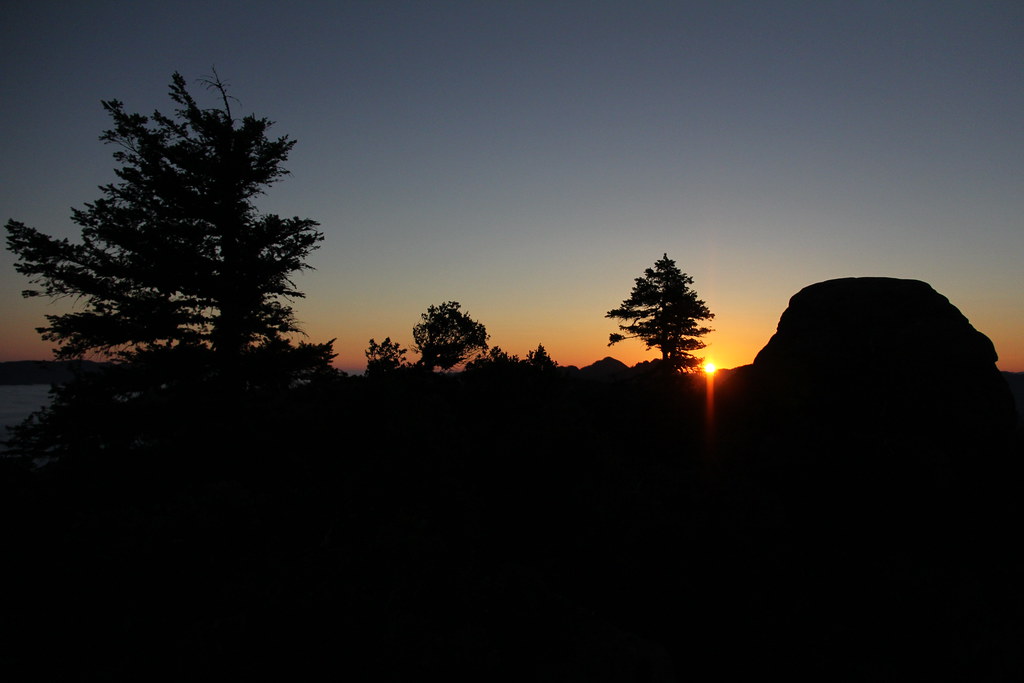In this striking evening scene, a serene forested landscape and rugged mountain terrain unfold as the sun sets, casting a dramatic golden and orange hue across the horizon. The sky transitions from a dark, clear blue at the top to lighter shades near the sun, which glows brightly amidst the treetops. The silhouettes of at least four trees, including two larger ones and two smaller trees or bushes, merge with the dark contours of large rocks and hills. A field extends in the background, its details obscured by the lack of ambient light. To the left, a faint outline suggests the presence of a lake or ocean, edged by a distant coastline. This composition creates a captivating contrast between the illuminated sky and the darkened terrestrial features, highlighting the calm beauty of twilight in this secluded, natural haven.